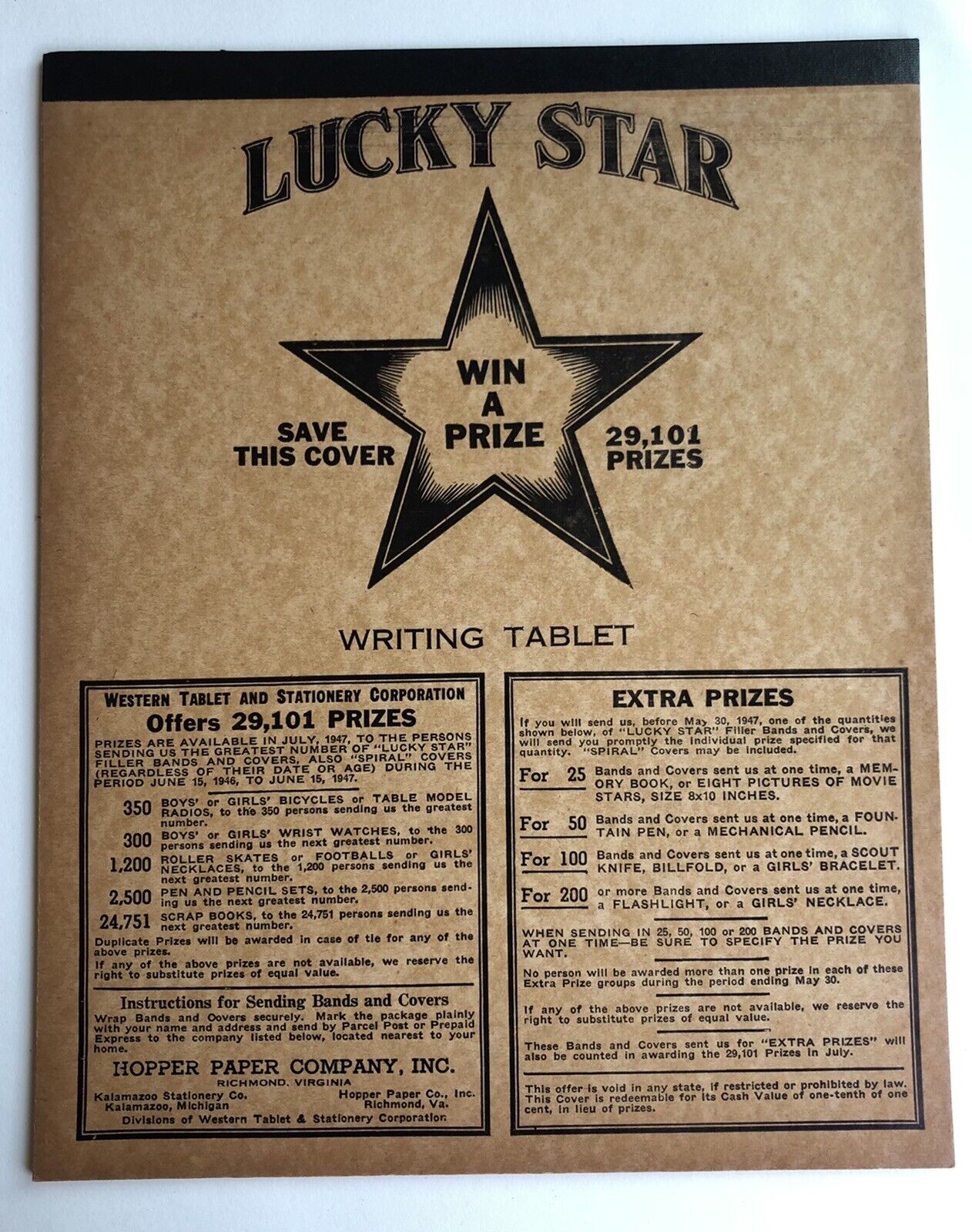This image features the back cover of a vintage writing tablet, likely from the mid-20th century, printed on beige parchment paper with black ink. At the top, a black banner or binding displays the phrase "Lucky Star" in block letters, arching slightly upward. Dominating the center is a large black star with a white center, where the words "Win a Prize" appear in black letters. Flanking the star, on the left it reads "Save this Cover" and on the right, "29,101 Prizes". Beneath the star, the text "Writing Tablet" is prominently displayed. The lower section of the cover contains two detailed informational boxes. The left box begins with "Western Tablet and Stationery Corporation offers 29,101 prizes", followed by fine print detailing prize listings and sponsorship from the Hopper Paper Company, Incorporated, along with affiliations to Richmond, Virginia, and Kalamazoo, Michigan. The right box highlights "Extra Prizes for 25, for 50, for 100, for 200" in similarly small print. This promotional cover is indicative of a contest aimed at children from past decades, featuring a nostalgic brown background.